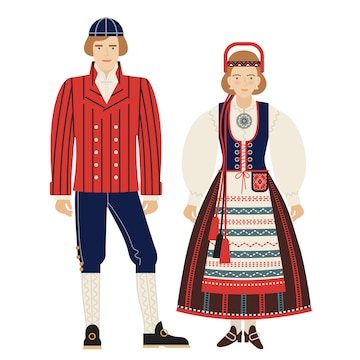The image features two animated characters, a man and a woman standing against a plain white background. The man, positioned on the left, is wearing an elaborate outfit that consists of a red jacket with vertical black stripes and ten white buttons, a white collared shirt underneath, and blue knickers that reach just below his knees. Completing his ensemble are long white socks, black shoes with gold accents, and a blue hat with white stripes. He has slightly longer brown hair that reaches his ears. 

On the right, the woman is dressed in a distinctive outfit reminiscent of Swiss or Dutch traditional attire. She wears a puff-sleeved white blouse under a black, blue, and red dress with white accents. The dress includes a blue vest section and a skirt with red and brown hues, finished off with black shoes and white socks or tights. Her headgear consists of a brown headband with a prominent red adornment, possibly resembling a handle, extending from the top. Both characters present an image suggestive of historical or cultural garb, further emphasized by their old-fashioned bob-style haircuts and the woman's corseted dress with an apron.